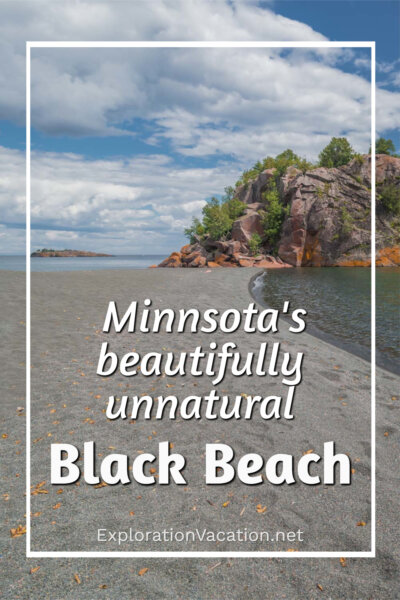The image captures a scenic beach on the left side, with dark green waters stretching to the right. In the background, a rocky, tree-covered mountain rises behind the beach, separated by the sea from a smaller mountain further in the distance. The sky is vibrant blue, scattered with multiple white clouds, suggesting a pleasant, clear day. The sandy beach area is sprinkled with yellow-orange leaves, adding a touch of autumn. Centrally embedded text reads, "Minnesota's beautifully unnatural black beach," highlighted within a white rectangular border. Below this, in smaller white-gray text, it says "ExplorationVacation.net," making it clear this is an advertisement for a travel site.